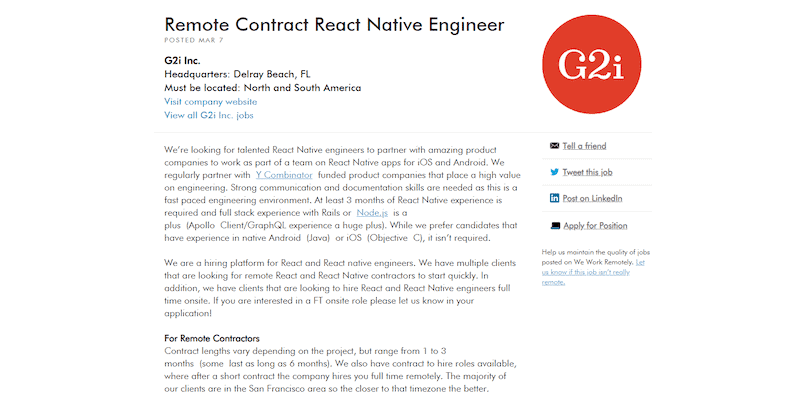**Job Posting: Remote React Native Engineer at G2i Inc**

G2i Inc, headquartered in Delray Beach, Florida, is seeking talented React Native engineers for remote contract positions. The company partners with premier product companies, including Y Combinator-funded enterprises, to develop high-quality iOS and Android applications.

**Key Responsibilities:**
- Collaborate with product companies and work as part of a team to develop React Native apps for iOS and Android.
- Maintain strong communication and documentation skills to thrive in a fast-paced engineering environment.

**Requirements:**
- Minimum of three months of experience in React Native development.
- Full stack experience with Rails or Node.js is advantageous.
- Experience with Apollo Client and GraphQL is highly desirable.
- Native Android (Java) or iOS (Objective C) experience is preferred but not mandatory.

**Opportunities:**
- G2i Inc offers multiple remote React and React Native contractor positions.
- Contract lengths vary from one to three months, with some extending up to six months.
- Full-time, onsite roles are also available. Interested candidates should indicate their preference in the application.
- Contract-to-hire roles are offered, where candidates may be hired full-time remotely after a short contract period.

**Location:**
- While the company's headquarters is in Florida, the majority of clients are located in the San Francisco area. Proximity to this time zone is beneficial.

For more information or to apply, visit the G2i Inc website and explore all available job opportunities. Join us and partner with amazing product companies to make a significant impact in the tech world.

**Contact:**
- G2i Inc Headquarters
- Delray Beach, Florida
- Visit G2i Inc's website for further details and application instructions.